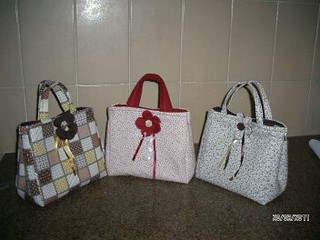The image is a small, low-resolution color photograph in landscape orientation with a barely discernible silver or white text label in the bottom right corner, traditionally where a date or time stamp might be found. It features a highly polished, dark gray marble kitchen countertop with a background of vertically oriented, light beige tiles separated by white grout. Arranged on the countertop in a semi-circle arc are three small handbags of a similar size but different styles.

The handbag on the left has a checkered pattern composed of white, black, yellow, pink, and gray squares, with a black flower and gold bow hanging down. Its short handle features the same checkered pattern. The central handbag is predominantly light pink with red speckles, featuring a red rose and two red strands hanging from the flower. It has a red handle. The right handbag is white with black speckles, adorned with a black button and silver hanging strings. Its handle mirrors the speckled pattern.